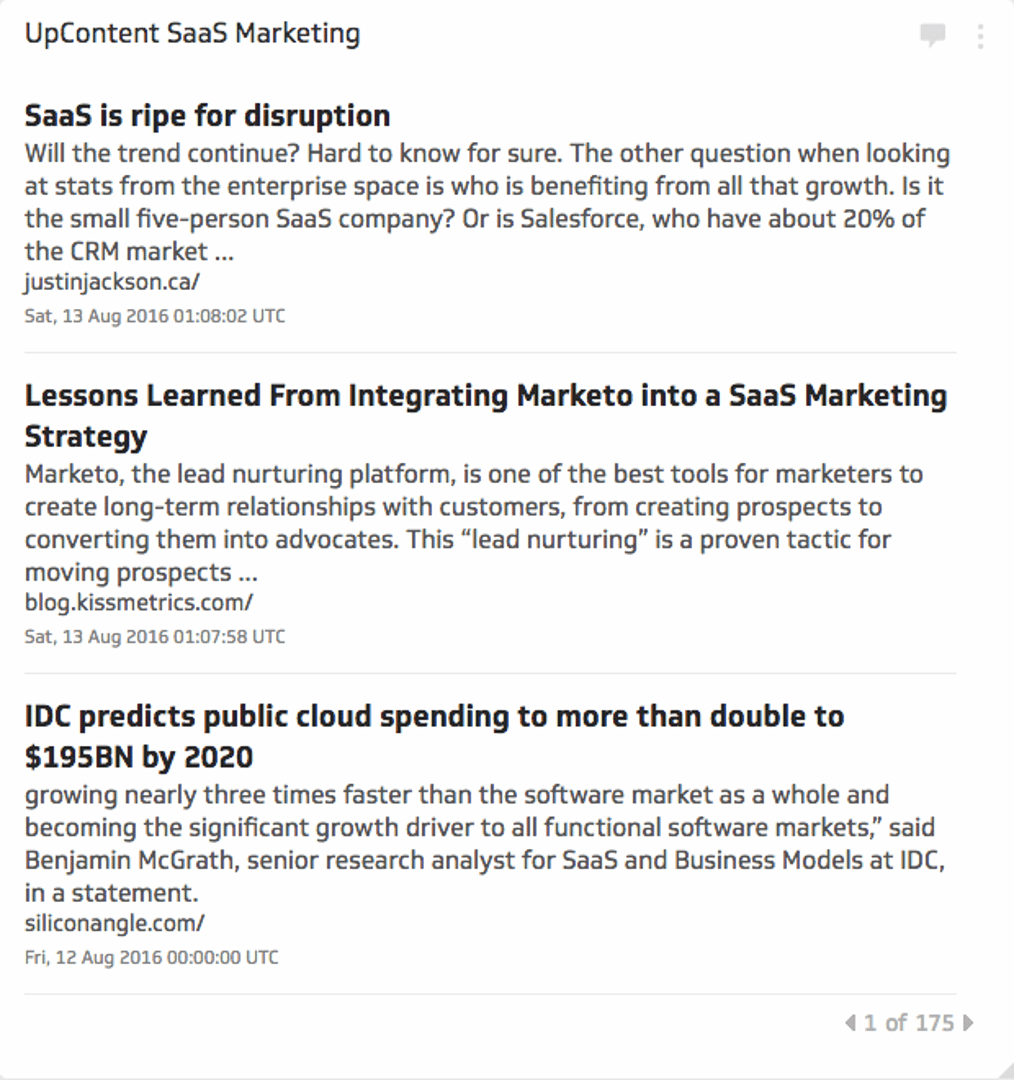Certainly! Here's a detailed, descriptive caption for the screenshot:

---

The image appears to be a screenshot from a feed reader displaying various articles related to SaaS marketing. The background is white with black text, and there are no images included. At the top, the text "SaaS Marketing" is prominently displayed, with the letters "S," "A," and "S" stylized as capital S, lowercase a, lowercase a, capital S.

The screenshot includes three distinct sections:

1. **First Section:**
   - **Title:** 
     "SaaS is ripe for disruption. Will the trend continue? Hard to know for sure."
   - **Content:** 
     This section explores the potential for disruption within the SaaS industry, questioning whether the trend will persist. It also examines who benefits most from the growth, comparing small five-person SaaS companies to giants like Salesforce, which dominates roughly 20% of the CRM market.
   - **Source:** 
     Justin Jackson's blog at justinjackson.ca.
   - **Publication Date:** 
     Saturday, August 13th, 2016 at 01:08:02 UTC.

2. **Second Section:**
   - **Title:** 
     "Lessons learned from integrating Marketo into a SaaS marketing strategy."
   - **Content:** 
     This segment highlights the benefits of using Marketo, a lead nurturing platform, in SaaS marketing strategies. It emphasizes Marketo's ability to foster long-term customer relationships, from prospect creation to conversion into advocates. The term "lead nurturing" is noted as a tried-and-true method for advancing prospects.
   - **Source:** 
     Blog at kismetrics.com.
   - **Publication Date:** 
     Saturday, August 13th, 2016 at 01:07:58 UTC.

3. **Third Section:**
   - **Title:** 
     "IDC predicts public cloud spending to more than double to 195 billion by 2020. I wonder if that actually happened."
   - **Content:** 
     IDC forecasts dramatic growth in public cloud spending, anticipating it will more than double to $195 billion by 2020, growing nearly three times faster than the overall software market. This growth is expected to drive significant advancements across all functional software markets, according to Benjamin McGrath, Senior Research Analyst for SaaS and Business Models at IDC.
   - **Source:** 
     SiliconANGLE.
   - **Publication Date:** 
     Friday, August 12th, 2016 at Midnight (00:00:00 UTC).

The screenshot indicates that this is page 1 of 175 available pages.

---